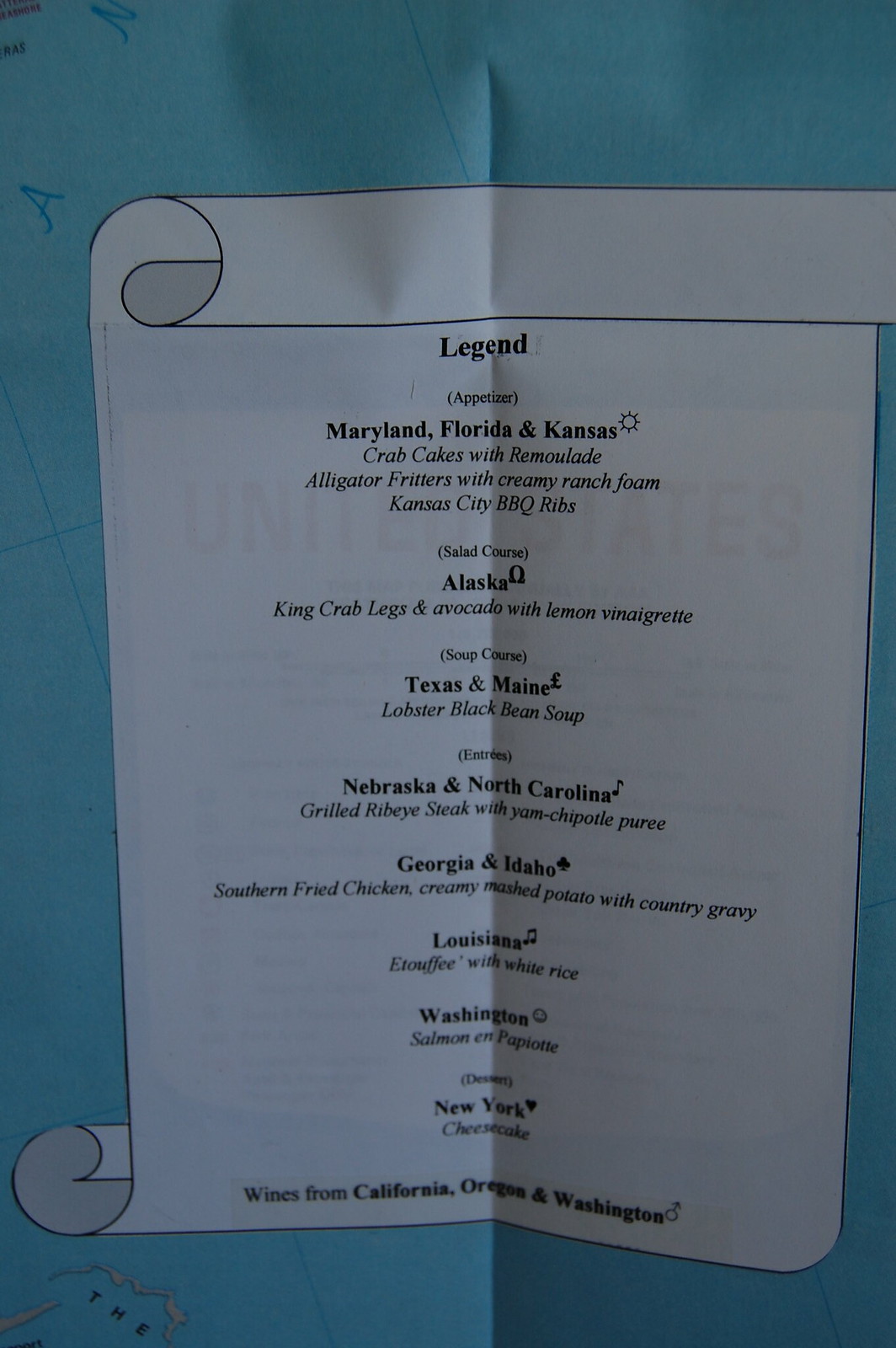The image features a menu with various regional dishes meticulously laid out in black text. At the top of the menu, the heading "Appetizers" introduces Maryland, Florida, and Kansas crab cakes with Rommel aid; alligator fritters with creamy ranch foam; and Kansas City barbecue ribs. Following this, the "Entrees" section features an array of delicacies, including grilled ribeye steak from Nebraska and North Carolina, accompanied by a chipotle purée; Georgia and Idaho fried chicken served with creamy mashed potatoes and country gravy; Louisiana étouffée with white rice; and Washington salmon en papillote. The "Desserts" section offers a classic New York cheesecake. 

The bottom of the menu highlights a selection of wines from California, Oregon, and Washington, with a male symbol positioned on the right. The background of the menu boasts a teal hue on the left and around the main areas, transitioning to a lighter blue along the outer edges, adding a calming aesthetic to the overall presentation.